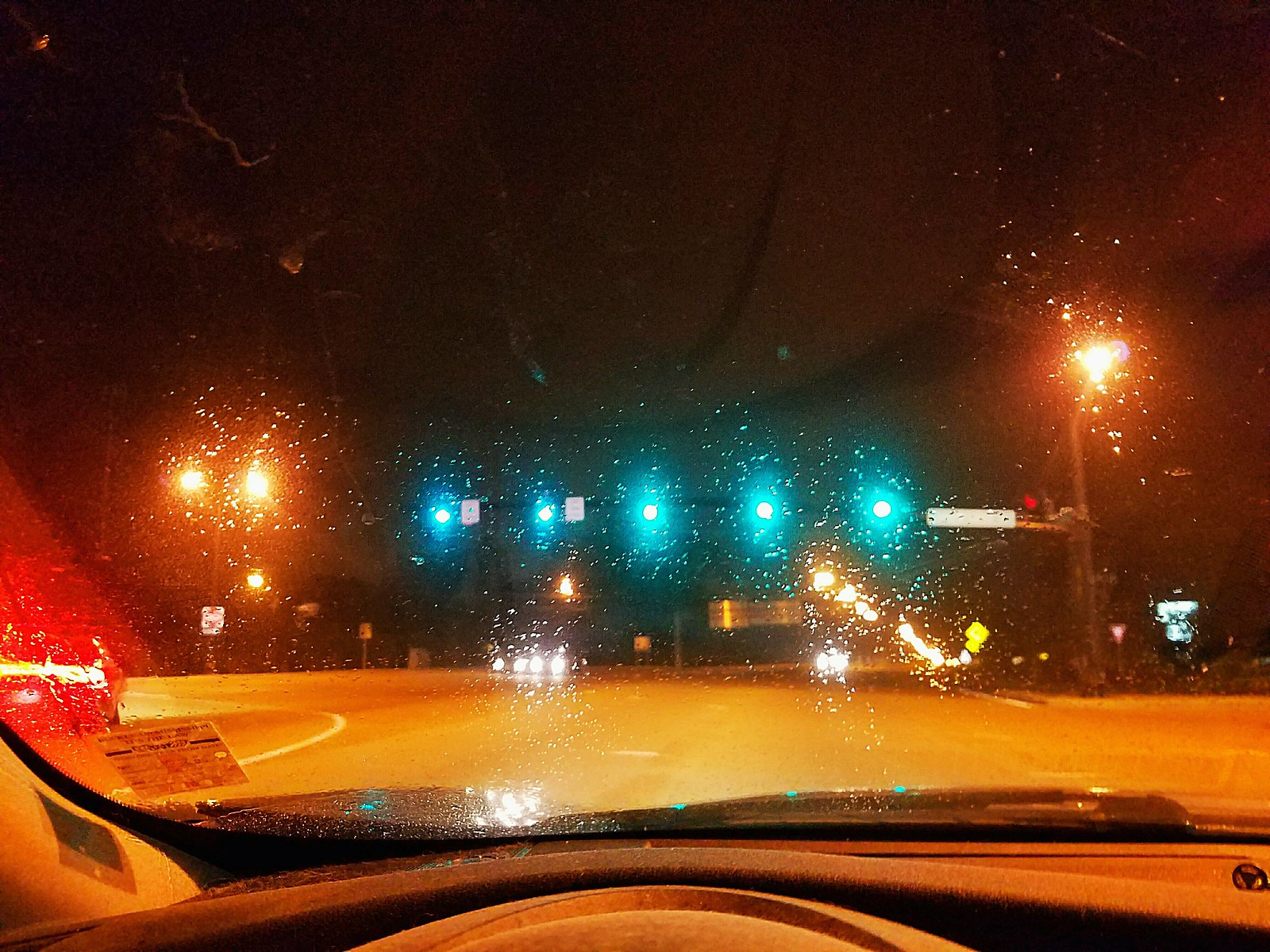Photographed from inside a moving car, this image captures a rainy street scene through the front windshield, which is speckled with raindrops that shimmer in the light. The wet road gleams under the glow of green stoplights, their reflections creating a vibrant, yet blurred, impressionistic image due to the motion. Street poles with attached traffic lights are visible both on the left and right sides of the road, contributing to the urban landscape. The car's black dashboard, adorned with a sticker, is prominently featured in the lower portion of the frame. To the left, a bright red light, possibly from another vehicle, stands out against the otherwise muted colors of the scene. Distant oncoming traffic is discernible by the white headlights piercing through the rainy haze. The overall atmosphere conveys a sense of motion and the relentless downpour of rain, evoking a quintessential rainy day commute.